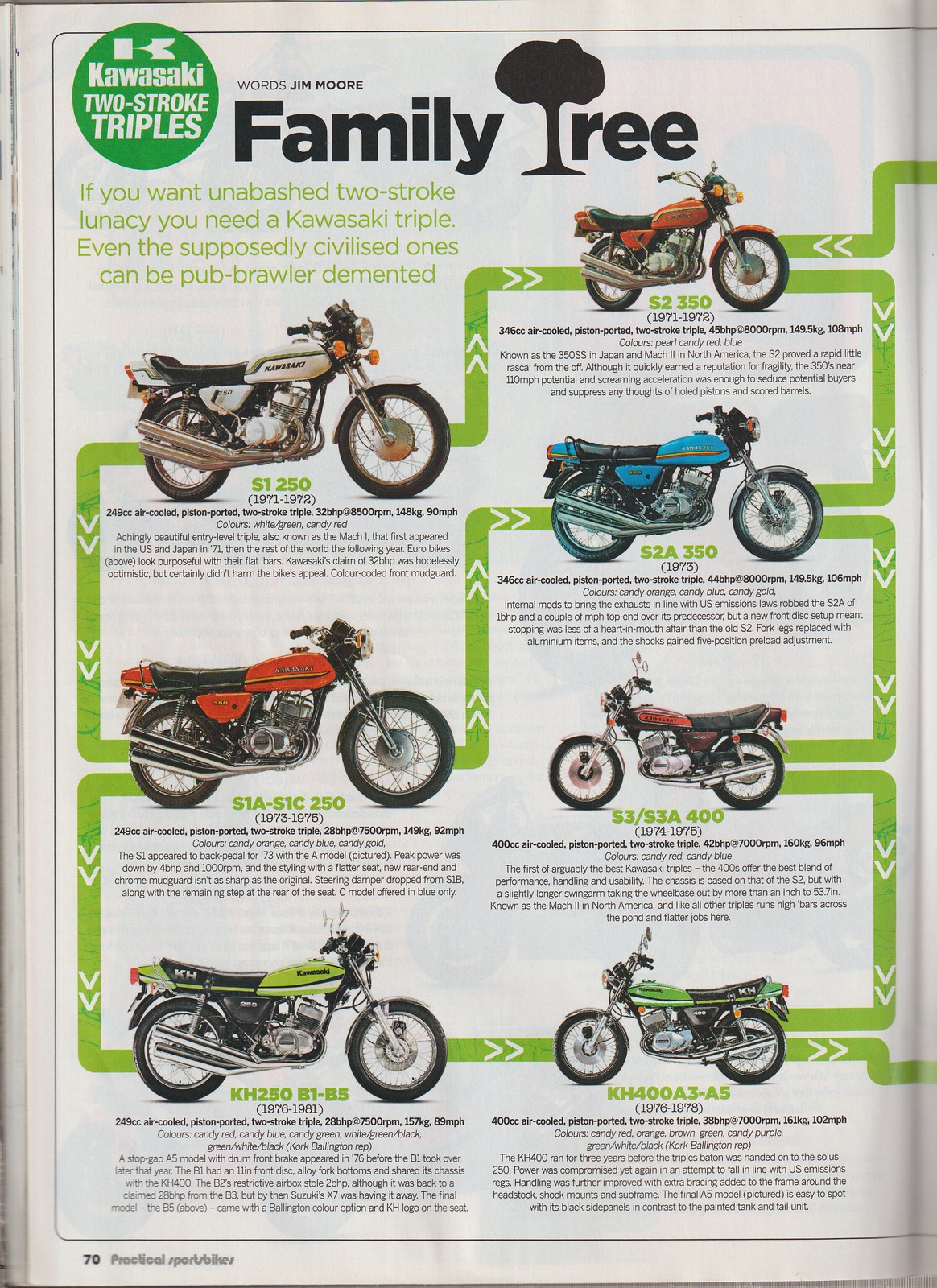The magazine page, likely from an issue focused on motorcycles, features a detailed advertisement for Kawasaki two-stroke triples. The layout consists of multiple elements: 

At the top of the page, there's a title "Family Tree," where the "T" is illustrated as a black tree drawing. Just above this title, the name "Jim Moore" is written. Positioned next to "Family Tree" within a green circle with white text, the letters "K" and the phrase "Kawasaki Two-Stroke Triple" appear.

Below the title, a prominent lime green caption reads, "If you want unabashed two-stroke lunacy, you need a Kawasaki triple. Even the supposedly civilized ones can be pub, brawler, demented." This is followed by a series of motorcycle images arranged in columns.

On the left column, three motorcycles are displayed, each with its respective details and prices in lime green, accompanied by smaller, difficult-to-read text beneath each bike. The motorcycles feature parts in various colors: one bike has red parts, another one is white, and a third one has blue parts.

On the right column, four more motorcycles are showcased, with similar layout and pricing in lime green, along with corresponding black text details. These bikes display parts in red, lemon, green, and once again, red.

Green lines with white arrows connect the images of the bikes, indicating a connection between them. The background of the page is white, with a reddish-gray tone typical of a magazine. In the bottom left corner, partially obscured, "70" is indicated as the page number along with "Practical Sports Bikes."

Overall, the magazine page portrays a captivating visual and textual presentation of Kawasaki's two-stroke triples, emphasizing their distinct characteristics and variety.